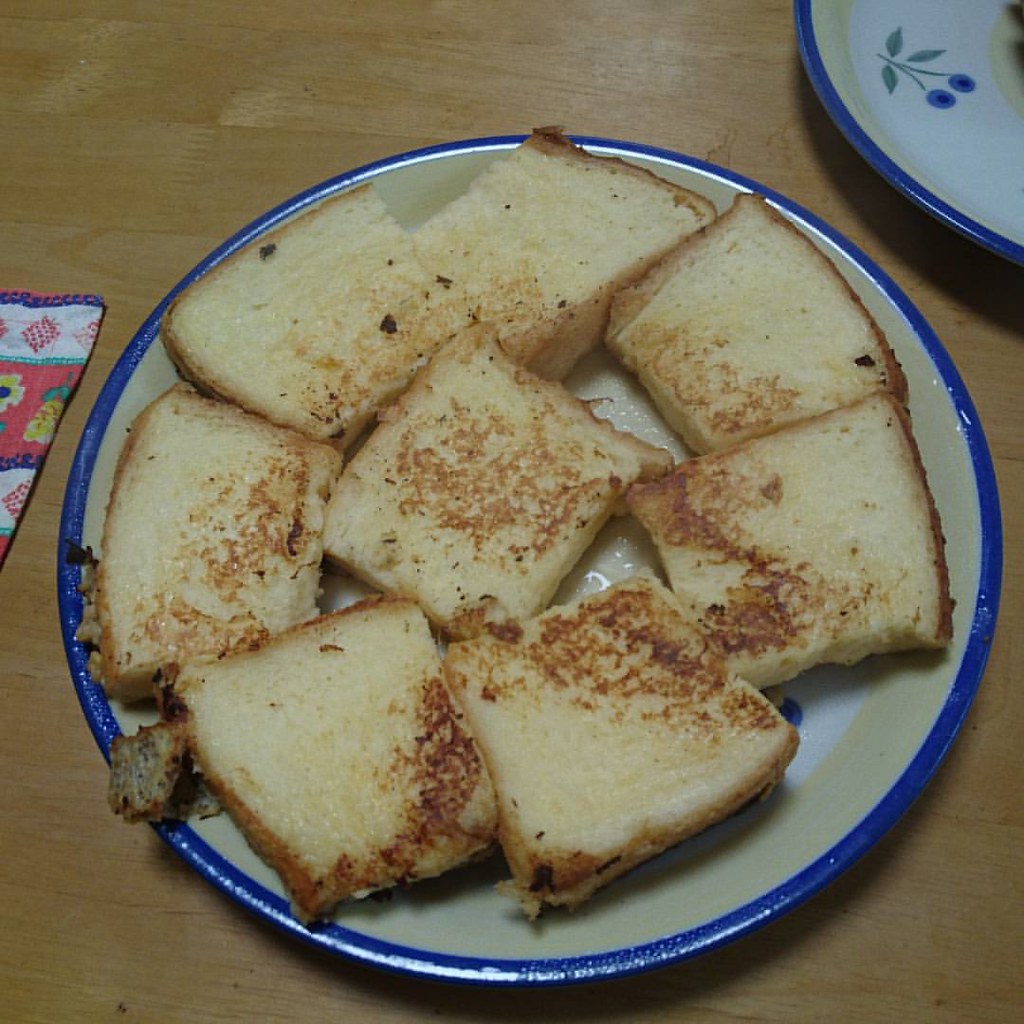The image features a vertical photograph of a circular plate of food resting on a natural blonde wood table. The plate has a distinctive design with a blue outer rim and a beige stripe on the inner rim, accompanied by small blue floral elements. Arranged neatly on the plate are eight perfectly grilled quarters of sandwich bread, golden brown in color, likely indicating they were grilled in butter rather than toasted. The slices form a ring with one piece in the center surrounded by seven others, all arranged flat without stacking. Visible in the top right corner is a portion of a matching plate, devoid of any food but featuring the same blue rim and floral design. Additionally, on the left side, a corner of a decorative napkin or placemat peeks into the frame, featuring a floral pattern in colors like white, coral, blue, green, and yellow. The overall composition of the elements, viewed from above, creates a detailed and inviting portrayal of the meal.